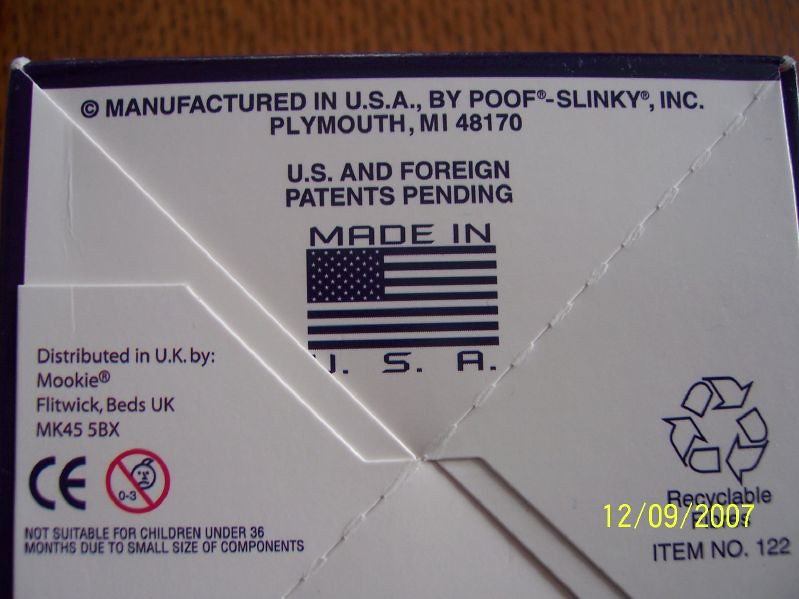**Image Description:**

The image depicts the underside of a product box. The box has a blue border around its white body. At the top of the box, the text reads: "AC manufactured in USA by Poof-Slinky, Inc." followed by "Plymouth, MI 48170". It also states: "US and foreign patents pending" and "Made in USA", accompanied by a small image of the USA flag.

On the left side, the text reads: "Distributed in UK by Mookie" followed by "Flitwick, Flitwick Beds, UK MK45 5BX". There are also various symbols including one with a "C" and an "E" and another depicting a red crossed-out baby head with "0-3" indicating that the product is not suitable for children under 36 months due to small components.

On the right-hand side, there's a recycling symbol with partially blocked text that appears to say "recyclable". Below this, the item number "122" is visible, but it, along with the recycling text, is partially obscured by a yellow date stamp: "12/09/2007".